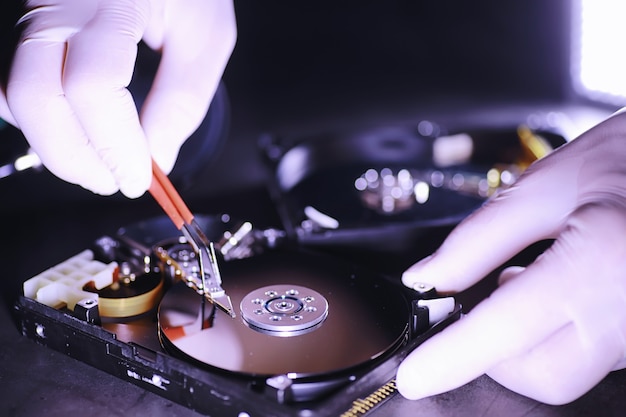This detailed color photograph captures an up-close shot of two hands, clad in white rubber gloves, meticulously working on a computer hard disk drive. The drive, housed in a flat black casing, has its cover removed, exposing the intricate inner components. The hands are seen using a pair of fine tweezers with an orange rubber handle and an angled head to manipulate the reader arm delicately. In front of a dark, cluttered workbench or machine shop area, illuminated by a bright light on the right, the image focuses sharply on the hands and the hard disk drive. To the right, the prominent black circular disk, resembling a record album or CD, is visible. Despite the out-of-focus background, which includes the top part of the drive, there is a sense of precision and attention to detail in the technician's careful work on the delicate electronic equipment.